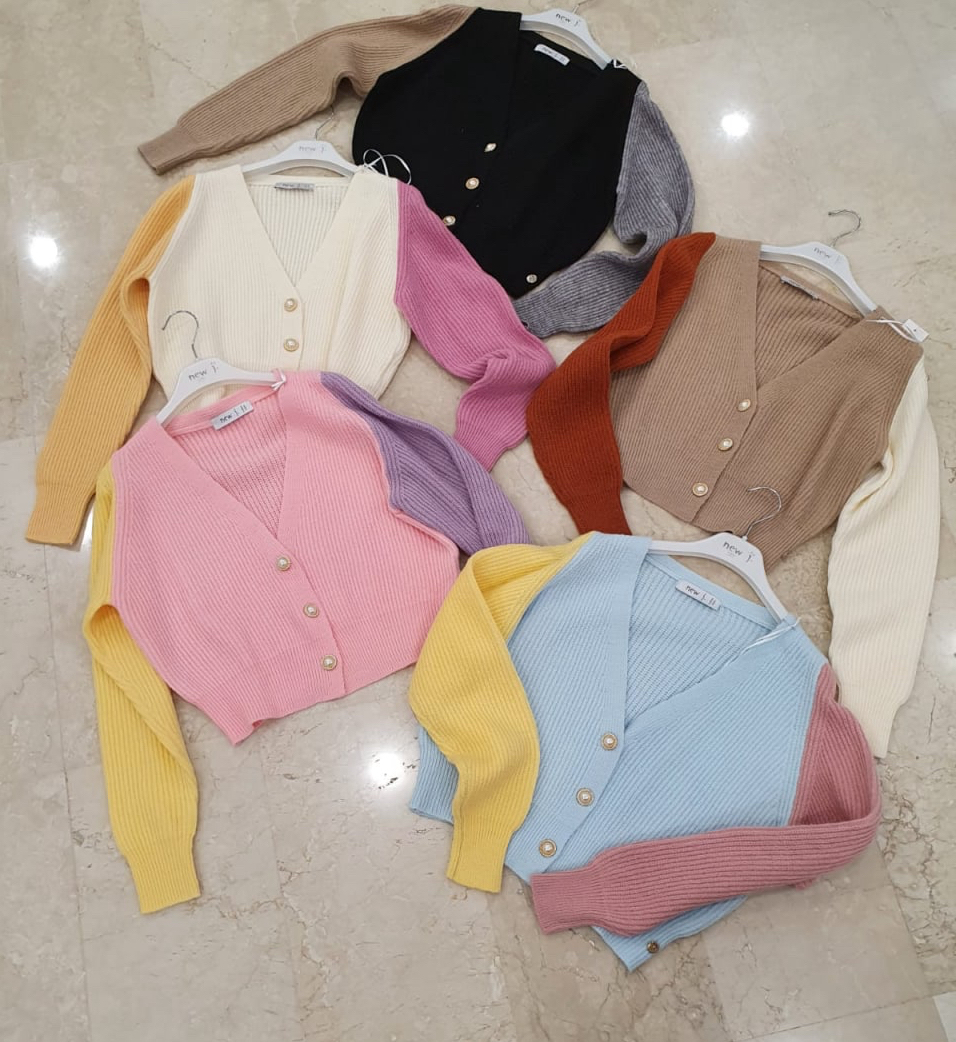The image depicts five women's long-sleeved tops laid out on a shiny, marble-like store floor, illuminated from above. Each top is hung on a white hanger and features a button-down vest in a different multicolored combination. The first top, situated at the bottom right, has a light blue vest with one yellow sleeve and one pinkish sleeve. Next to it is a pink vest top with a yellow sleeve and a purple sleeve. Above this is a white vest top with a brownish sleeve and a pinkish sleeve. To the right of this is a brown vest top with a darker brown sleeve and a white sleeve. The final top, positioned at the top of the arrangement, is a black vest with a gray sleeve and a brown sleeve. All the tops are partially overlapping but clearly visible against the smooth, stone-like floor.